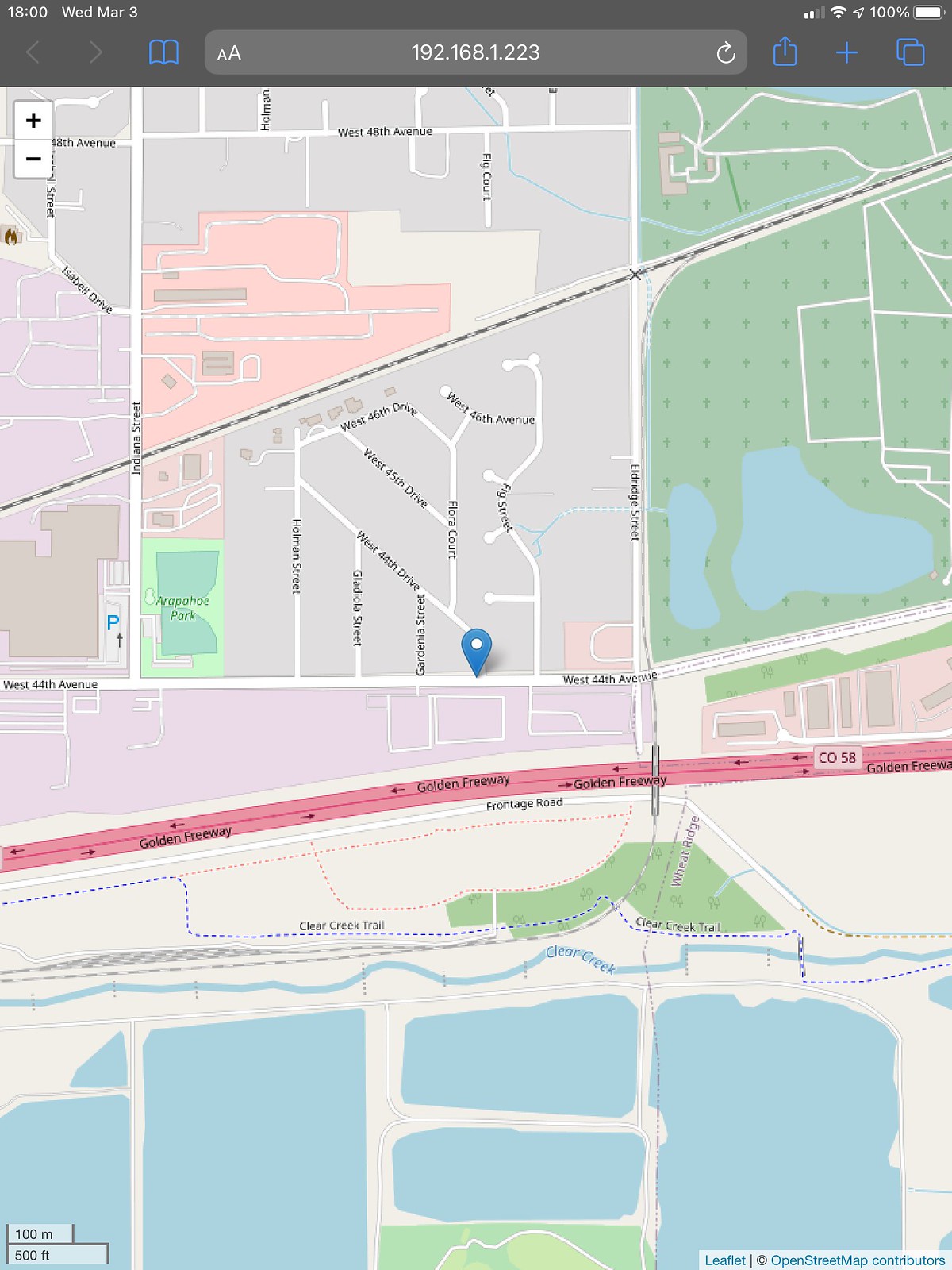This image displays a digital map, likely captured as a screenshot from a cell phone with a visible search bar at the top containing the code “192.168.1.223”, possibly an IP address or coordinate. The map highlights a residential neighborhood with a blue pin featuring a white dot securely placed at the center, marking a specific location.

The top 10% of the image is reserved for the search bar. Below this, the map is predominantly segmented into various land and water areas. At the bottom of the map, water bodies are neatly divided into four horizontal segments. Above these, a stream runs across the lower portion of the screen, separating the water segments from a green area.

Further up, a red highway, labeled “C-O-58”, likely indicating Colorado Route 58, traverses horizontally across the map. Above this highway is a predominantly residential zone illustrated in shades of pink and gray, segmented by numerous roads. On the left side of this area is a park, with its name partially obscured, starting with the letter “A”.

On the right-hand side, beyond CO-58, there is a mix of pink residential areas and another expansive green zone. This green area features two small ponds near its lower part and a larger pond near its upper part. Scattered within this green region are small dots arranged in horizontal and vertical alignments, possibly indicating features or pathways within the area.

Overall, the detailed map clearly delineates various residential, recreational, and infrastructural elements, offering a comprehensive view of the neighborhood and its notable landmarks.